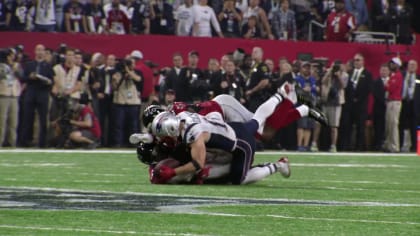The photo captures a dynamic scene from a football game, showcasing an intense moment where four players are piled on the ground, each fighting for possession of the ball. The players' jerseys display a mix of red, white, gray, and blue, without any visible text or numbers. Three players are face down, and one is face up, potentially having the ball. The backdrop includes a red wall, a line of officials, cameramen, and spectators along the sidelines. Fans in the stands are visible in the top right, all standing and cheering. The field features green turf and a partially visible blue and white logo, possibly belonging to the New England Patriots. Overall, the image vividly conveys the excitement and chaos typical of football tackles.